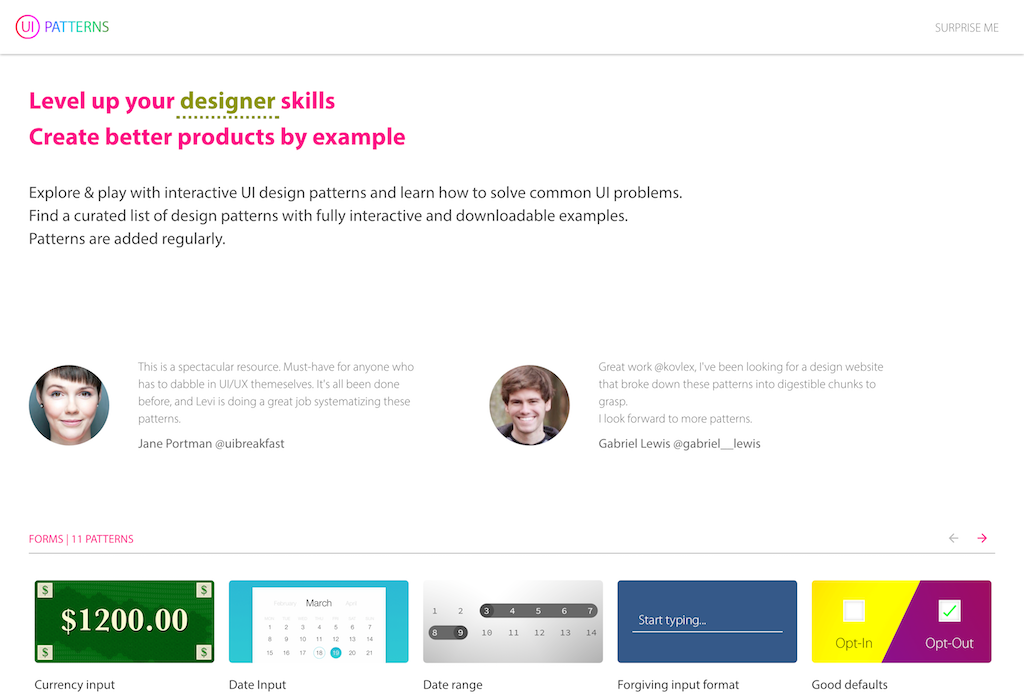This screenshot showcases a website called UI Patterns. The logo features the letters "UI" encased in a vibrant red and purple gradient circle, with the text similarly styled in a gradient. Adjacent to the logo, the word "Patterns" is displayed with a multi-colored font: the "P" in purple, "A-T" in blue, "T-E-R-N" in green, and the "S" in brown. To the far right, the words "Surprise Me" appear in transparent gray text. Both the logo and the "Surprise Me" text are underscored by a transparent gray line.

Beneath the header, a title invites users to "Level up your designer skills, create better products by example." Most of the text is in purple, except for the word "Designer," which stands out in green and is underlined with a dotted line. 

Following this, a caption encourages users to "Explore and play with interactive UI design patterns and learn how to solve common UI problems. Find a curated list of design patterns with fully interactive and downloadable examples. Patterns are added regularly."

Below this, two reviews are prominently displayed. Jane Portman of UI Breakfast praises the resource, describing it as "a spectacular resource, a must-have for anyone who has to dabble in UI/UX themselves. It's all been done before, and it's doing a great job systemizing these patterns." Gabriel Lewis, identifiable by his handle @Gabriel_Lewis, adds, "Great work at Covlex. I've been looking for a design website that broke down these patterns into digestible chunks. I look forward to more patterns."

Further down, a bar labeled "Forms" displays 11 design patterns. It includes five distinct boxes, such as:
- A $1,200 bill graphic labeled "Currency Input."
- A March calendar labeled "Date Input."
- A non-specific calendar showing the days 1 through 14 with a range highlighted from 3 to 9, labeled "Date Range."
- A search bar prompting users to "Start typing," labeled "Forgiving Input Format."
- A segment with two options: "Opt-In" in a yellow box and "Opt-Out" in a purple box, with "Opt-Out" being checked, labeled "Good Defaults."

Each element on the screenshot is meticulously organized to ensure clear navigation and understanding of the UI Patterns website's offerings.